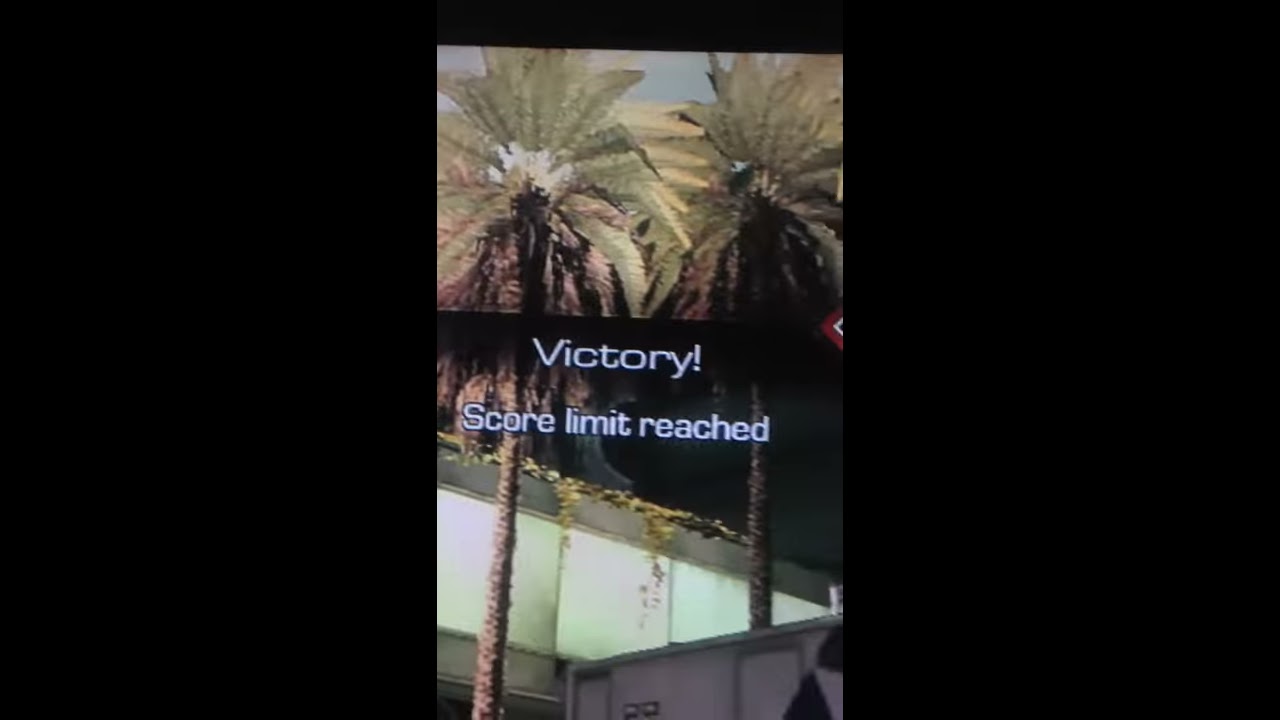The image is a vertically oriented screenshot set against a pitch-black background, divided into three vertical sections where only the middle section contains a picture. The middle section is a digital, somewhat pixelated scene likely from a video or computer game. The scene shows the exterior of a building with a light green central wall flanked by grey-painted top and bottom portions. In the foreground, two palm trees with green and brown dried leaves stand tall, their stems brown. Behind the trees, the sky is a bluish-grey. White text is superimposed at the top of the image, stating "Victory! Score limit reached." The overall photo quality is not very high, giving it a pixelated and digital appearance.